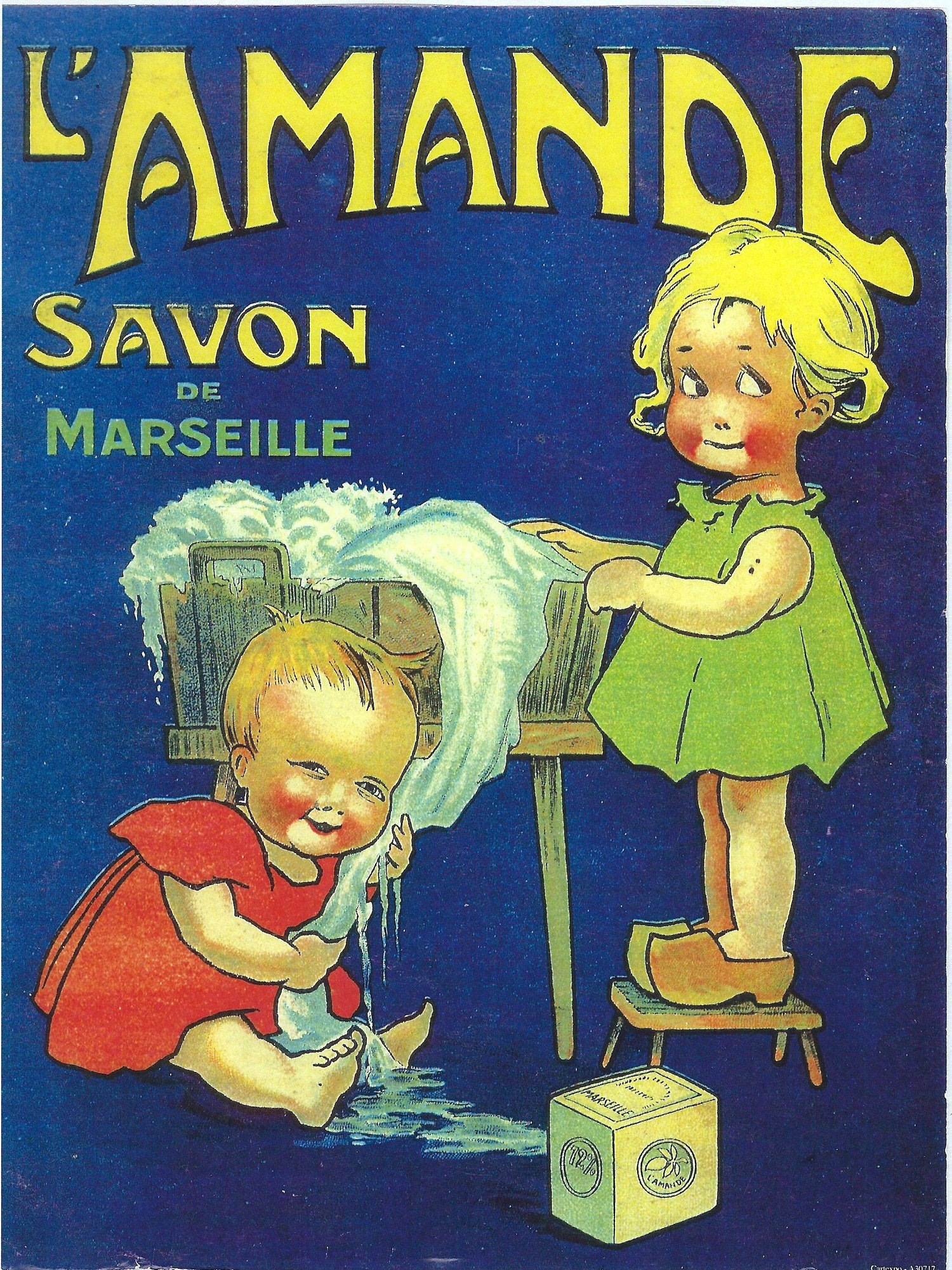This vintage Art Nouveau style advertisement, possibly from the 1930s or 40s, depicts a charming scene centered around almond soap. Against a dark blue background with stylized yellow lettering that reads "Le Monde Savant de Marseille," the illustration showcases two blonde-haired children engaged in washing clothes. A young girl, dressed in a green dress and wooden clogs, stands on a short wooden stool beside a wash basin, her hands immersed in the water. Below her, a baby, wearing a yellow dress, sits on the floor, laughing joyfully while holding onto a piece of wet clothing, seemingly taken from the basin. At the baby's feet sits a box of the almond soap, reinforcing the product being advertised. This classic Art Nouveau poster combines vibrant colors and intricate details to evoke a nostalgic and familial atmosphere.